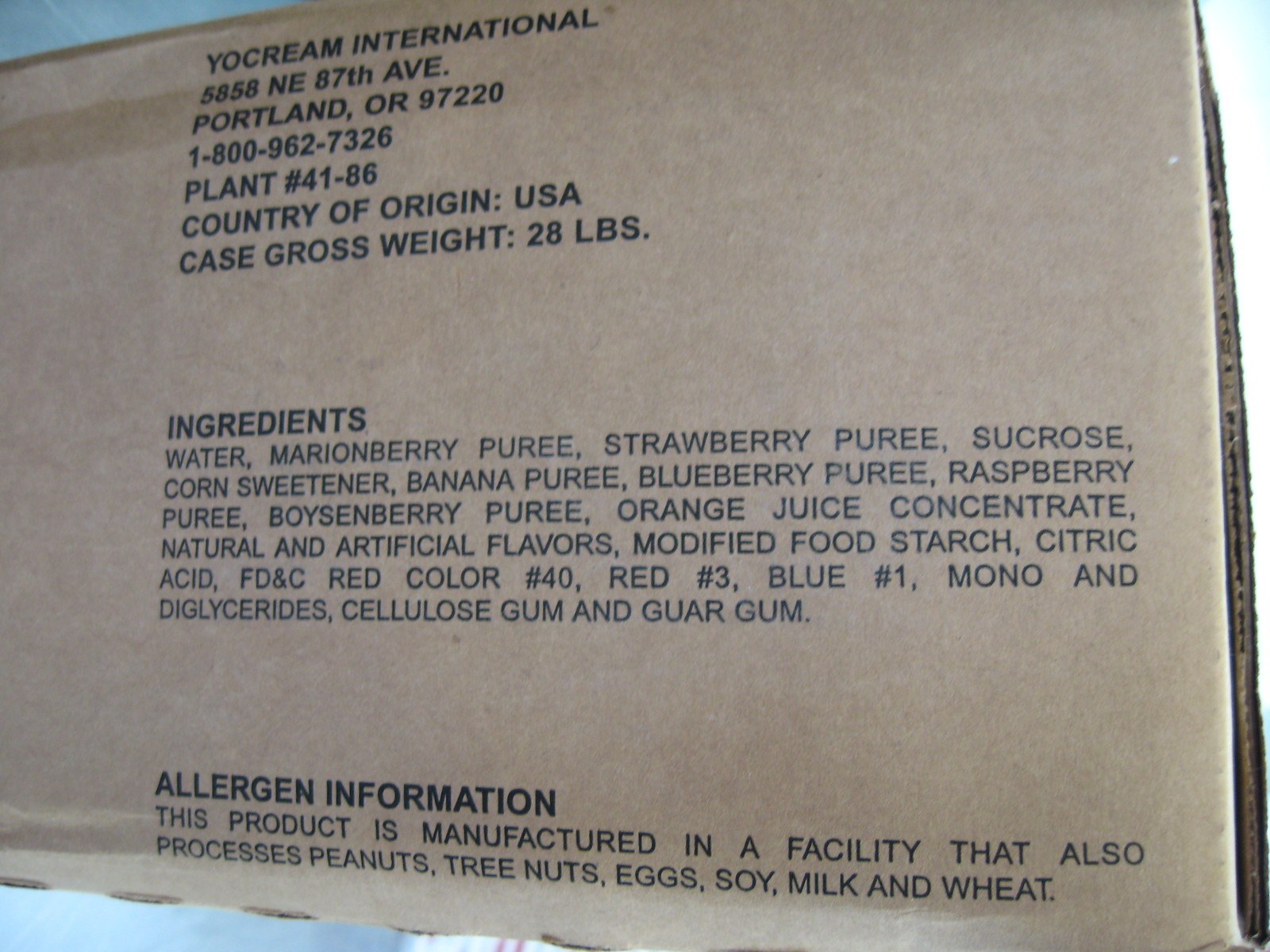This is a detailed description of a bulk product packaged in a plain, light tan brown cardboard box with black text. The box, which appears to be used for commercial purposes, is labeled with "Yocream International" and the address "5858 Northeast 87th Avenue, Portland, Oregon 97220." A contact phone number "1-800-962-7326," as well as plant number "41-86," are also provided on the box. The product's country of origin is the USA, with a case gross weight of 28 pounds.

The ingredients list includes a variety of fruit purees and additives: water, marionberry puree, strawberry puree, sucrose, corn sweetener, banana puree, blueberry puree, raspberry puree, boysenberry puree, orange juice concentrate, natural and artificial flavors, modified food starch, citric acid, FD&C red color numbers 40 and 3, blue color number 1, monoglycerides and diglycerides, cellulose gum, and guar gum. The product comes with an allergen warning, stating that it is manufactured in a facility that also processes peanuts, tree nuts, eggs, soy, milk, and wheat.